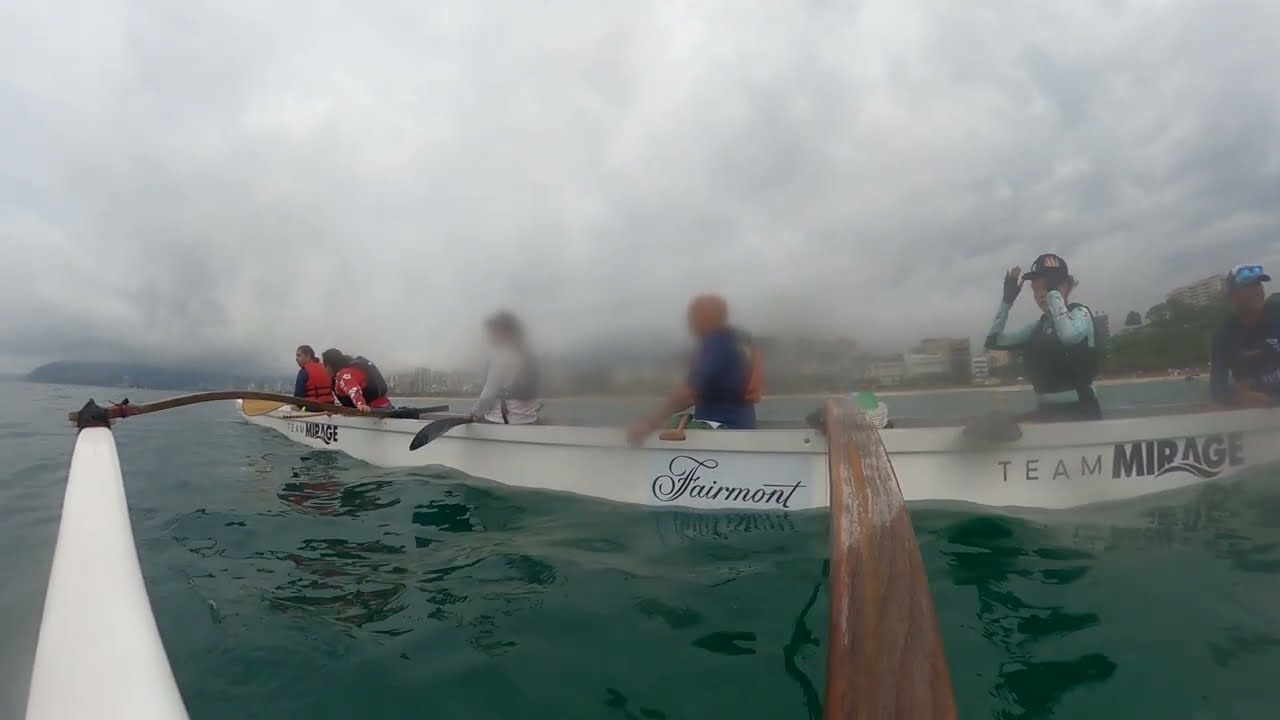This image depicts a long, thin rowing boat with six people onboard, situated on a calm, dark aqua-blue water surface. The boat, identified as "Team Mirage" in black, thin letters on a white hull, features the word "pheromone" in elaborate script at the center. At the stern, a person in a light blue long-sleeved shirt, potentially wearing a darker life vest, and a distinctive red hat with a white dot, gazes out to the side, holding the brim of their hat.

Adjacent to them, another individual, bald and dressed in a short-sleeved black shirt, grips the side of the boat. Moving forward, one teammate, partially obscured by thick grayish clouds, wears light gray clothing and maneuvers an oar. Another crew member, draped in dark clothes with yellow and red accents, similarly leans over the boat, while the fifth visibly sports a red life jacket over dark long sleeves and utilizes another wooden oar.

The background blends foggy skies and thick clouds with distant green-covered mountains, contributing to an overall sense of impending rain. Shadowy reflections of the rowers on the boat ripple in the water below. A serene shoreline dotted with blurred buildings and foliage is faintly discernable under the dense cloud cover, emphasizing the remote and mist-laden setting of this competitive rowing scene.